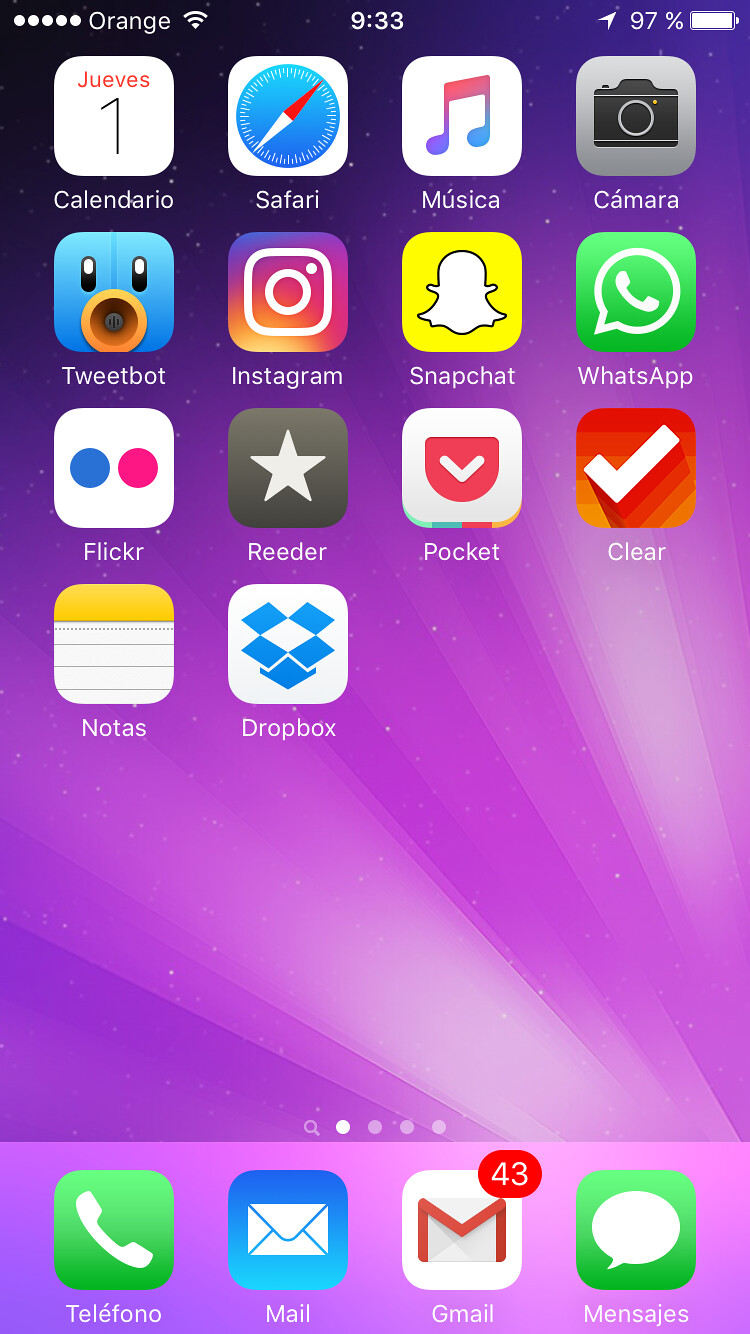The image depicts a screenshot of a cell phone's home screen, likely belonging to a Spanish-speaking user. At the very top, five small dots are visible, followed by text that reads "orange." Adjacent to it is a Wi-Fi connection symbol. Centrally located at the top is the time, displayed as 9:33, and at the far right is the battery icon indicating a 97% charge.

The home screen features several app icons arranged in a grid. The apps include Colanderio Safari (the browser), Musica, Camera, Tweetbot, Instagram, Snapchat, WhatsApp, Flickr, Reader, Pocket, Clear, Note, Tareas (tasks), and Dropbox. Each app is accompanied by its distinctive logo. The wallpaper background is a gradient of different shades of purple.

Below the app icons, there are four small dots and a magnifying glass icon, indicating multiple home screens, with the first dot highlighted. At the very bottom of the screen are four primary app icons: Telefono (displayed with a green square and a white phone symbol), Mail (depicted with a white envelope on a blue background), Gmail (which shows 43 unread messages), and Messages (for text messaging).